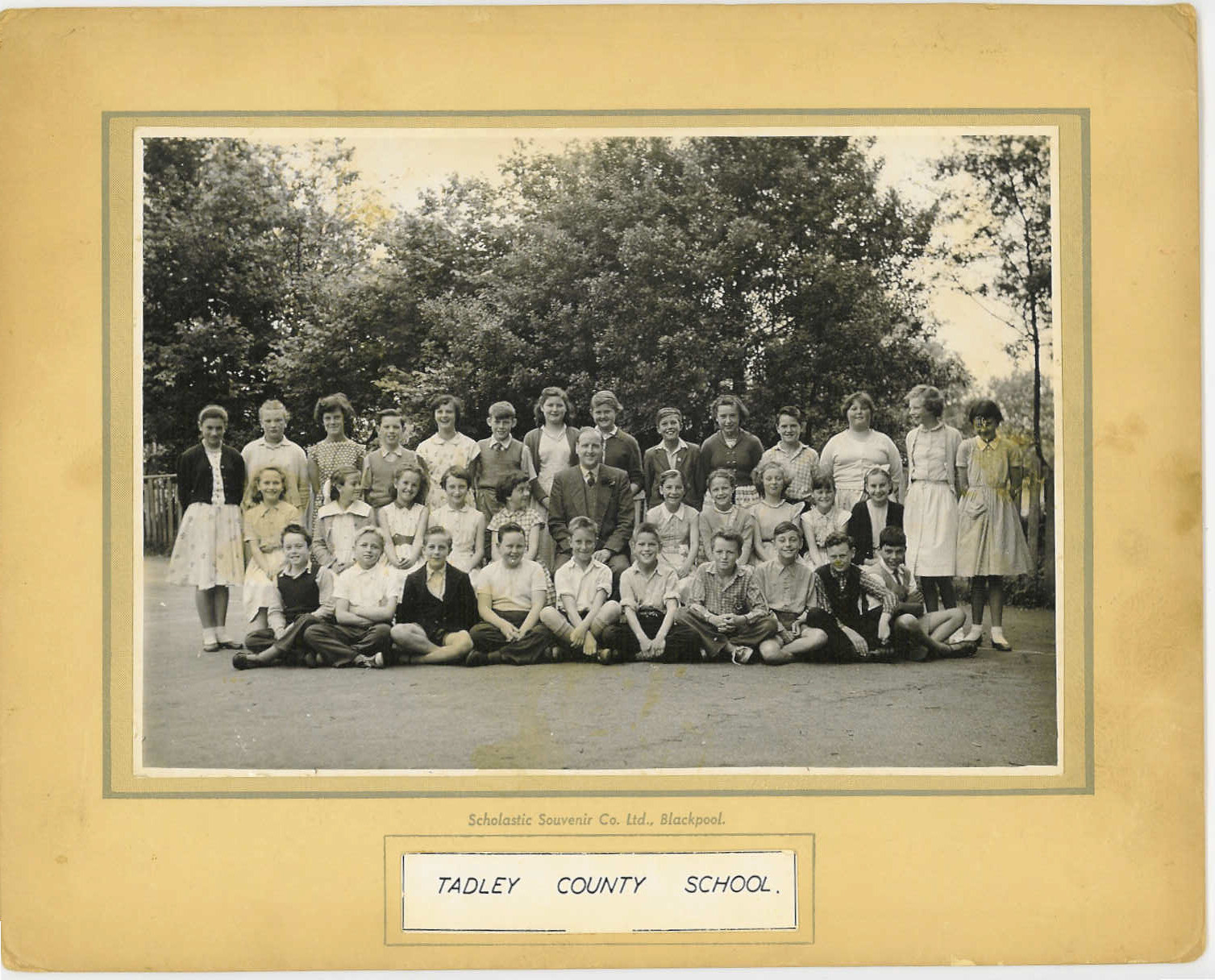This image is a sepia-toned, class group photo of students from Tadley County School. The photo, which shows signs of aging with slight coloration issues and stains, is bordered by a yellowed frame with a thin gray line encircling it. Notably, the bottom of the frame has "Tadley County School" written in white, and "Scholastic Souvenir Company LTD Blackpool" inscribed in black. 

In the picture, there are three rows of children, appearing to range in age from 8 to 14 years old. The first row has children sitting on the ground in a cross-legged (Indian-style) posture. The second row consists of children sitting in chairs, while the third row has older children, predominantly girls aged 12 to 14, standing. In the center of the group is a man presumed to be the principal or another school official, wearing a business suit complete with a vest and tie, appearing to be around 50 years old. Behind the group, a few trees can be seen against the sky, suggesting an outdoor setting. The children are smiling and looking attentively at the camera, capturing a moment of their shared school experience.